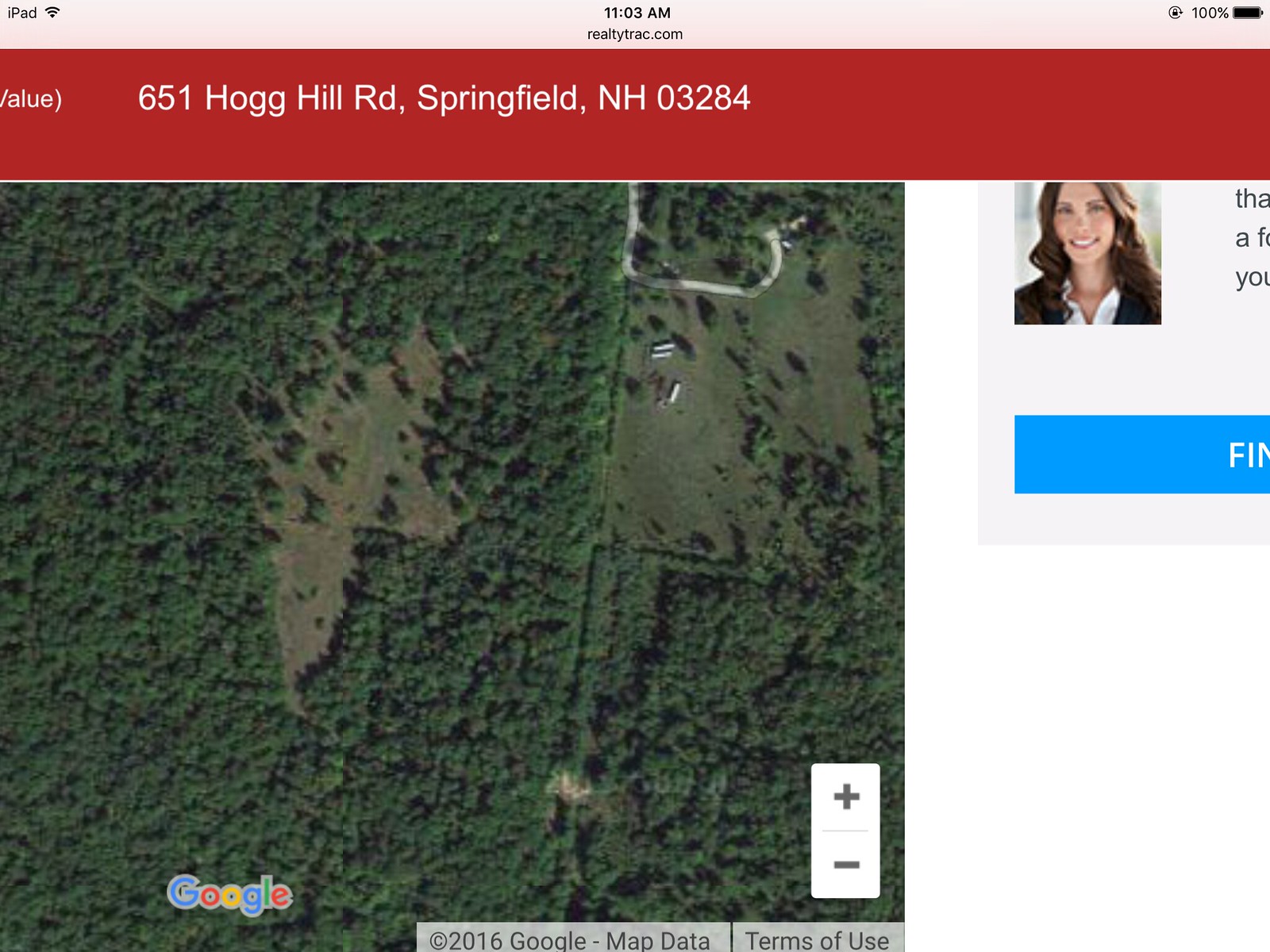This is a detailed screenshot taken from an iPad, indicated by the "iPad" label and Wi-Fi symbol in the upper left, with a full battery icon at 100% and a lock symbol encircled in the upper right. The time displayed on the iPad is 11:03 AM, and the web page on view is from RealtyTrack.com. The main visual content is a Google Maps image dating back to 2016, displaying the address 651 Hog Hill Road, Springfield, New Hampshire, 03284 in a prominent red banner with white text at the top.

The map reveals an overhead view of a predominantly green, wooded area with patches of grassland. Towards the upper right of the map, there is a white, hook-shaped road, alongside which three small objects, likely buildings or trailers, are positioned on the grass. The lower portion of the screen includes the colorful Google logo and notes on the map data and terms of use. To the right of the red banner, there's a professional photograph of a young Caucasian woman with long brown hair, presumably the real estate agent based on the website context. Additionally, there are map navigation tools such as a white portrait rectangle with plus and minus signs located on the lower right, used for enlarging or shrinking the map view.